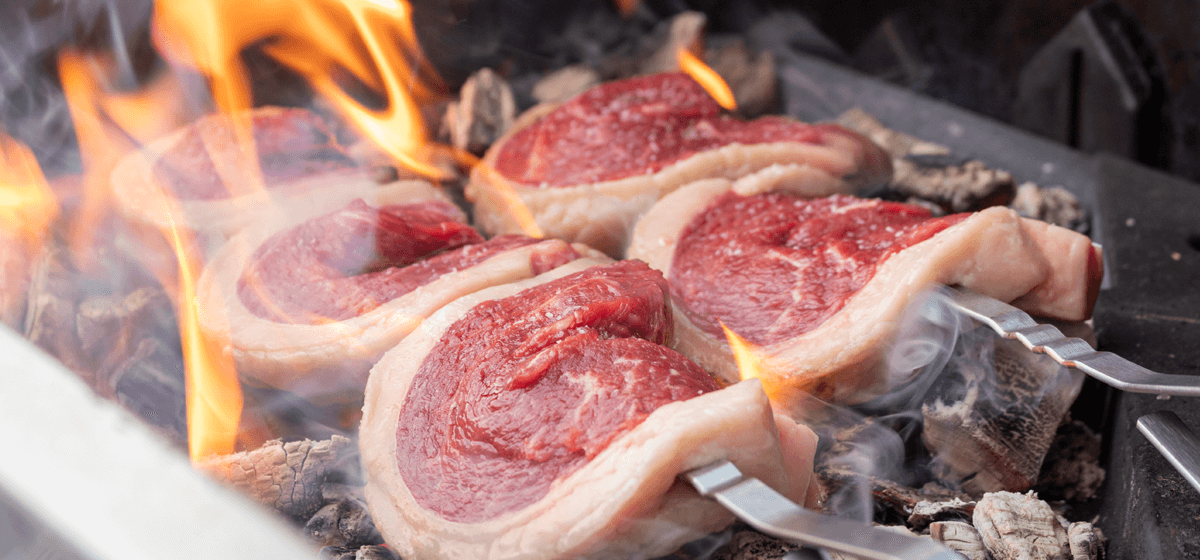A photograph captures at least five large, semi-circular cuts of meat, likely pork, being smoked. The fatty outer layer of the meat is reminiscent of light human skin, while the interior remains a bright red, indicating freshness. The meat is positioned directly against smoldering wood chips and coals within a trough-like enclosure, which emits visible flames, particularly toward the back left and front sections. Metallic or aluminum straps are used to hold the meat in place over the heat source, ensuring thorough cooking as the flames and heat interact intimately with the meat. The scene vividly portrays a rustic and intense smoking process, with the gleaming flames and rich colors of the meat providing a striking contrast.